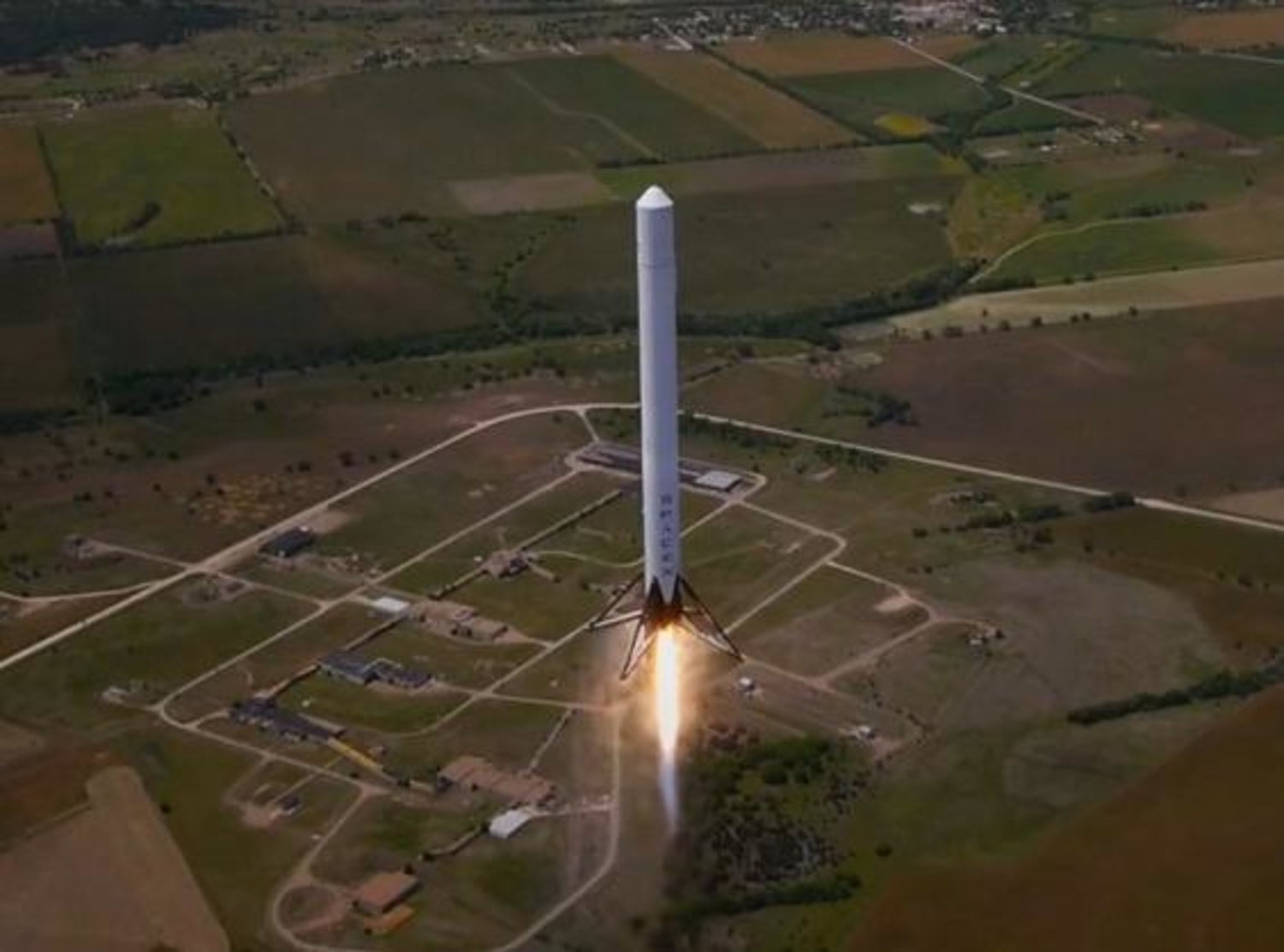The image captures a dramatic aerial view of a white, cylindrical SpaceX rocket either preparing to launch or already in flight, with golden flames jetting from its base. The rocket features a pointed, somewhat triangular tip and stabilizing fins at the bottom. It is seen soaring above a patchwork of green farmland, dotted with trees, roads, and buildings. The daytime setting illuminates the scene, highlighting the varying shades of green grass and the well-defined patches of farmland below. The image is taken from a high vantage point, possibly from a tower, an airplane, or a high mountain, providing a clear and expansive view of the landscape stretched out beneath the ascending rocket.